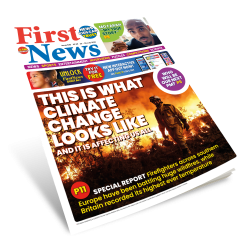The front page of the "First News" newspaper features a vivid and dramatic design. At the top, "FIRST" is prominently displayed in bold red text, followed by "NEWS" in striking blue text. On the right-hand side, there's an image of a man with a mustache and goatee, although the specifics about who he is remain unclear.

The main headline dominating the page reads, "THIS IS WHAT CLIMATE CHANGE LOOKS LIKE AND IT IS AFFECTING US ALL," in bright white, bold uppercase letters. The accompanying image underlines the urgency of the headline: a firefighter is captured walking away from a wildfire-ravaged forest, with intense oranges, yellows, and whites painting a harrowing backdrop of flames. 

Below the headline, within a yellow circle marked with a "P" and the number "11," there's an inscription that reads, "SPECIAL REPORT." The text further elaborates in white, emphasizing that firefighters across southern Europe have been combating expansive wildfires, while Britain registered its highest-ever temperatures. However, the remaining text about the firefighter is in yellow, and is relatively small and blurry, making it challenging to decipher completely.

Overall, the newspaper's layout is colorful but somewhat cluttered with attention-grabbing elements, making some of the smaller text difficult to read.